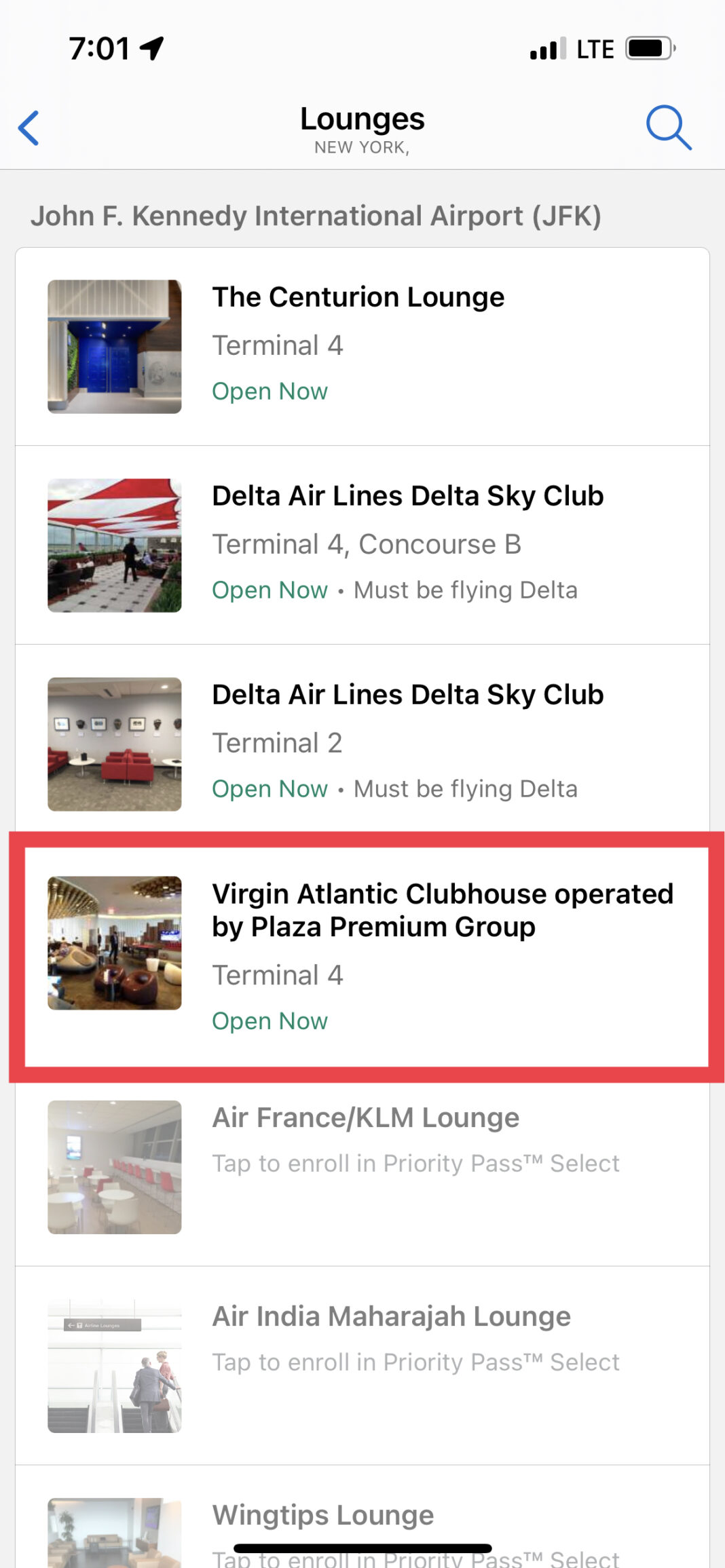This screenshot appears to be taken from either a tablet or a cell phone. At the very top of the screen, the time is displayed as 7:01, though it doesn't specify whether it is AM or PM. To the right of the time, the LTE network signal strength is shown with three out of four bars, and the battery icon indicates a charge level of approximately three-quarters full.

Below this top bar, there is a blue arrow pointing to the left, suggesting a back option. In the center, the word "Lounges" is prominently displayed in black text with "New York" written beneath it. On the far right, there is a magnifying glass icon, likely representing a search function.

Moving further down, the user is shown options related to John F. Kennedy International Airport (JFK), indicated by the text "John F" followed by "John F Kennedy International Airport" in full, with "JFK" in brackets. It is clear that the user is searching for lounges at JFK airport.

The first option listed is the Centurion Lounge located in Terminal 4, which is currently open. A small photo snippet of either the lounge entrance or interior accompanies this listing.

Below this is the listing for the Delta Airlines Delta Sky Club in Terminal 4, Concourse B, also marked as open now, with a similar photo snippet. Another Delta Sky Club lounge is listed next, this time in Terminal 2, and it is also open.

The currently selected lounge is the Virgin Atlantic Clubhouse operated by Plaza Premium Group, located in Terminal 4. This listing stands out with a thick, bold red outline.

Following this are further lounge options: the Air France KLM Lounge, the Air India Maharaja Lounge, and the Wingtips Lounge, each accompanied by a small image preview. All lounges are noted as being open. This comprehensive list suggests the user is comparing different lounges available at JFK airport.